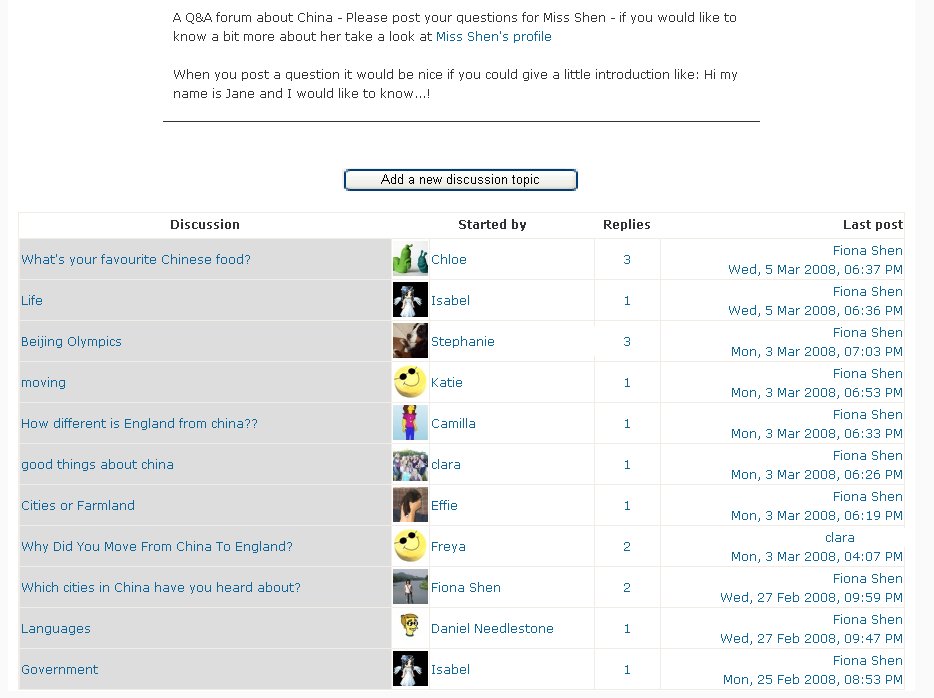**Detailed Caption:**

This screenshot captures a Q&A forum dedicated to inquiries about China, designed for users to post questions specifically for Ms. Shen. At the top, it prominently reads "A Q&A forum about China. Please post your questions for Ms. Shen." There's an invitation to learn more about Ms. Shen via a linked profile. Users are encouraged to introduce themselves with prompts like "Hi, my name is Jane and I would like to know..."

Beneath the introductory text, there is a noticeable button labeled "Add a new discussion topic." The forum is structured into four columns: "Discussion," "Started By," "Replies," and "Last Post." Under "Discussion," the exact topic is displayed. "Started By" includes the user’s chosen icon or image and their name. "Replies" counts the number of responses, and "Last Post" provides the responder's name along with the day of the week, date, and time of their last post.

For instance, the first discussion topic reads, "What's your favorite Chinese food?" initiated by Chloe, who has a corresponding icon. It shows that there are three replies, with the last post by Fiona Shen on Wednesday, 5 March 2008, at 6:37 PM. Other posted questions include "How different is England from China?," "Why did you move from China to England?," and "Which cities in China have you heard about?" Contributors to these questions include Isabel, Effie, and Stephanie. Most replies, varying from one to three per topic, are predominantly from Fiona Shen, dating from 25 February 2008 to 5 March 2008.